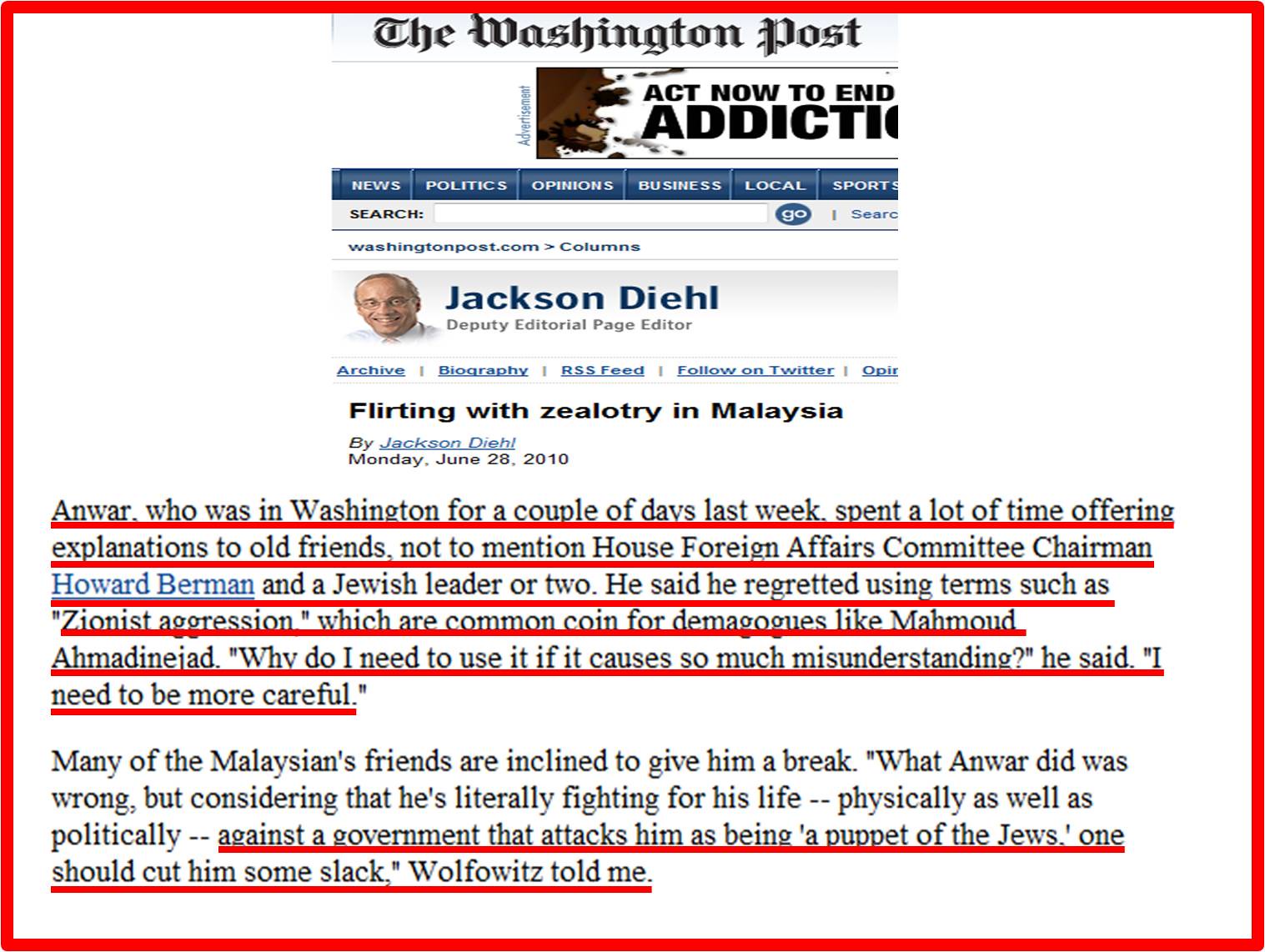This is a detailed screenshot of a Washington Post article titled "Flirting with Zealotry in Malaysia" by Jackson Diehl, dated Monday, June 28, 2010. The image features a white background with black text prominently underlined in red, presumably to emphasize certain phrases. At the top, there is a picture of the editor, Jackson Diehl, whose name is displayed. The article discusses Anwar, who recently spent time in Washington explaining himself to old friends and key figures such as House Foreign Affairs Committee Chairman Howard Berman and a few Jewish leaders. Anwar expresses regret for using inflammatory terms like "Zionist aggression," commonly used by demagogues like Mohammadinejad, and acknowledges the need to be more careful with his words. The article notes that many of Anwar's Malaysian friends are sympathetic, given his dire political and physical situation, and quotes Wolfowitz suggesting that Anwar deserves some leniency due to the relentless government attacks portraying him as a puppet of the Jews. The overall layout suggests that the snapshot was taken from the Washington Post's website.